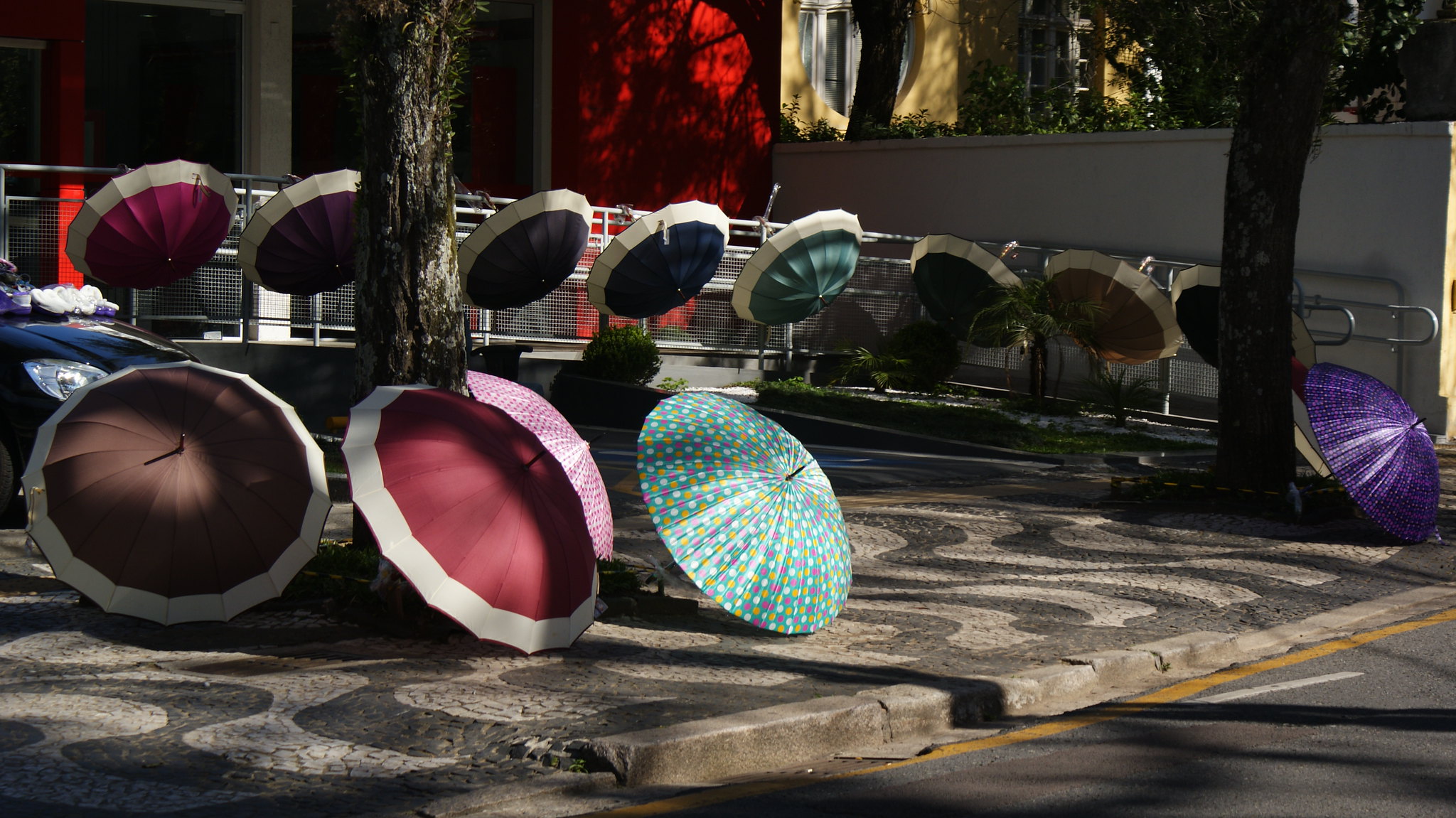The image captures a vibrant, eclectic collection of 11 open umbrellas, artistically arranged on a stone pavement with a wavy, curvilinear design. The umbrellas, in an array of colors and patterns including brown, cherry red, pink, blue with floral designs, green, orange, and purple, are spread out across a sidewalk-esque area that transitions into a courtyard near a car park. Some umbrellas are leaning against a sleek silver railing, while others are dispersed around tree trunks and lying on the shaded ground, implying the presence of numerous trees above. In the background, a striking red building is separated from a yellow house by a visible fence, complementing the lively, multi-hued scene below. The entire scene exudes a whimsical charm, with the diverse umbrellas creating a feast of colors against the urban landscape.